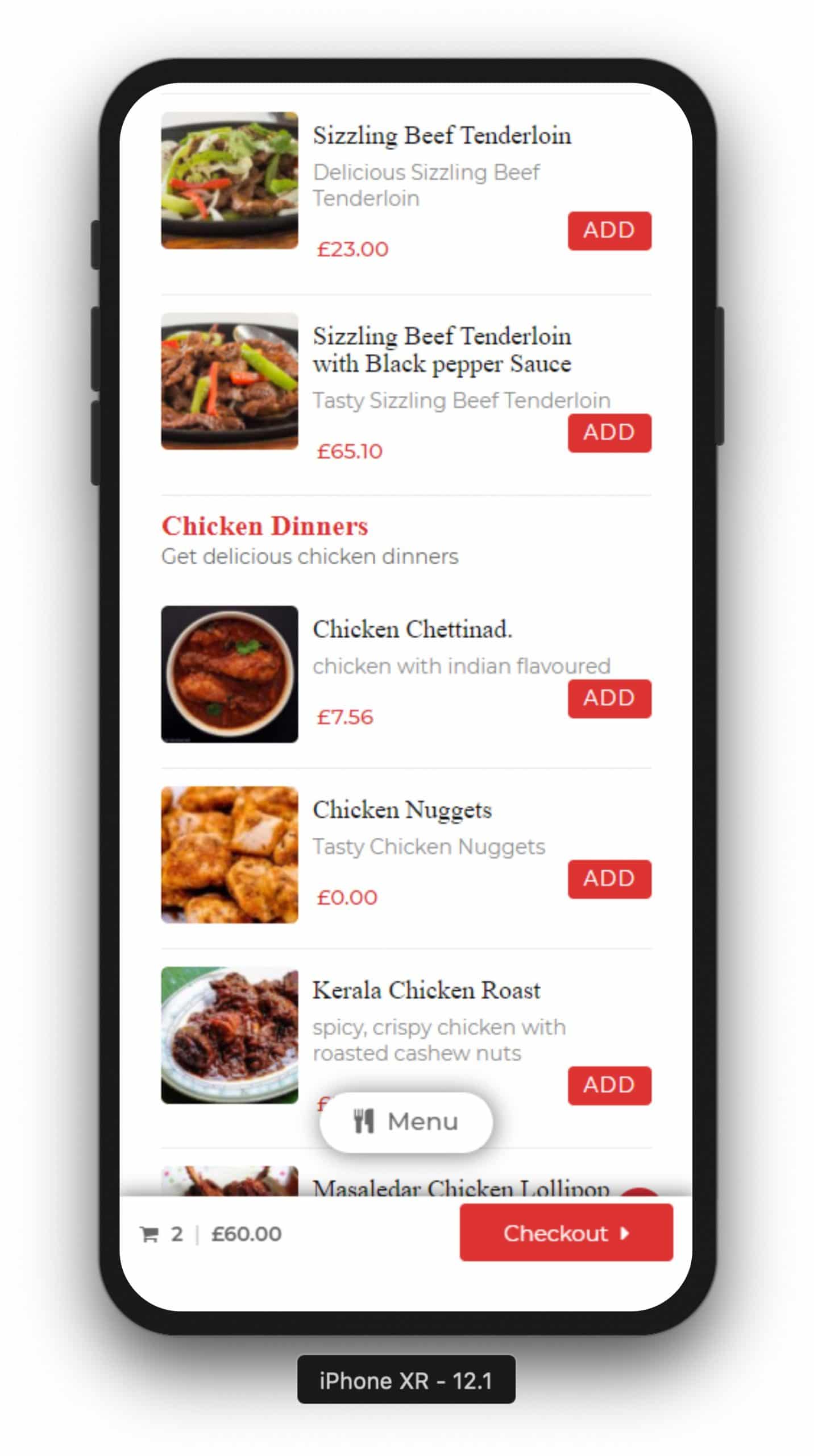The image is a screenshot from a restaurant menu, showcasing various dishes on a clean, white background. Each item is accompanied by prices and an "Add" button in bright red. The first featured dish is "Sizzling Beef Tenderloin," priced at £23, which appears smaller in portion compared to its variant, "Sizzling Beef Tenderloin with Black Pepper Sauce." The latter is described as a larger, more steak-heavy dish, priced at £65.10. 

Following the beef dishes, the menu presents a variety of chicken options. There are "Chicken Dinners," including a "Chicken with Indian Flavors" priced at £7.56, and "Chicken Nuggets" listed with a zero price, potentially indicating a special offer or error. Additionally, there's a "Perla Chicken Roast," described as spicy and served with roasted cashew nuts, though its price is obscured by a selection box labeled "Menu." 

The screenshot also reveals that two items have already been added to the cart, totaling £60. The checkout button, prominently displayed in red, is available for finalizing the order.